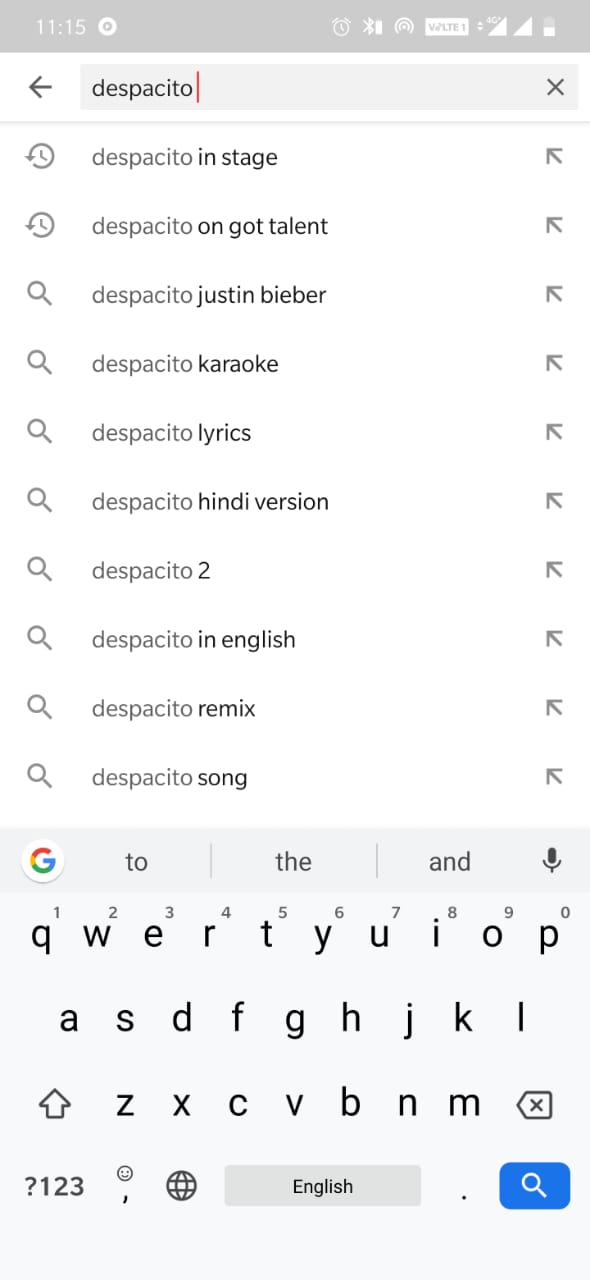**Detailed Caption:**

The image displays a screenshot with a grey background and white text reading "1115" at the top. Below this, there are two concentric circles. On the right-hand side of the screen, icons indicate various statuses: an alarm clock icon, a Bluetooth symbol, a battery icon positioned oddly near the Bluetooth symbol, a sun icon, and indicators reading "LTE 1" and "4G" alongside another cellular status icon and a half-filled battery icon.

In the main section of the screenshot, a white background features a black arrow pointing left at the upper left corner, next to a grey search box containing the word "Desperado." A black "X" is situated in the right-hand corner of this search box. Below are search history suggestions including "Desperado on stage," "Desperado on Got Talent," followed by autocomplete suggestions: "Desperado on Jeff Beaver," "Desperado on Karaoke," "Desperado Lyrics," "Desperado Hindi Edition," "Desperado 2," "Desperado English," "Desperado Remix," and "Desperado Song."

At the bottom of the screenshot, a QWERTY keyboard is displayed on a white background with black text. The top row of the keyboard includes the numbers 1-9 and 0 in the upper right corner, highlighted in grey. Below the keyboard, there is a row that switches to a numeric keypad, features a question mark, numbers 1, 2, 3, a smiley face icon, a globe icon, the text "English," a period key, and a blue search button with a white magnifying glass icon.